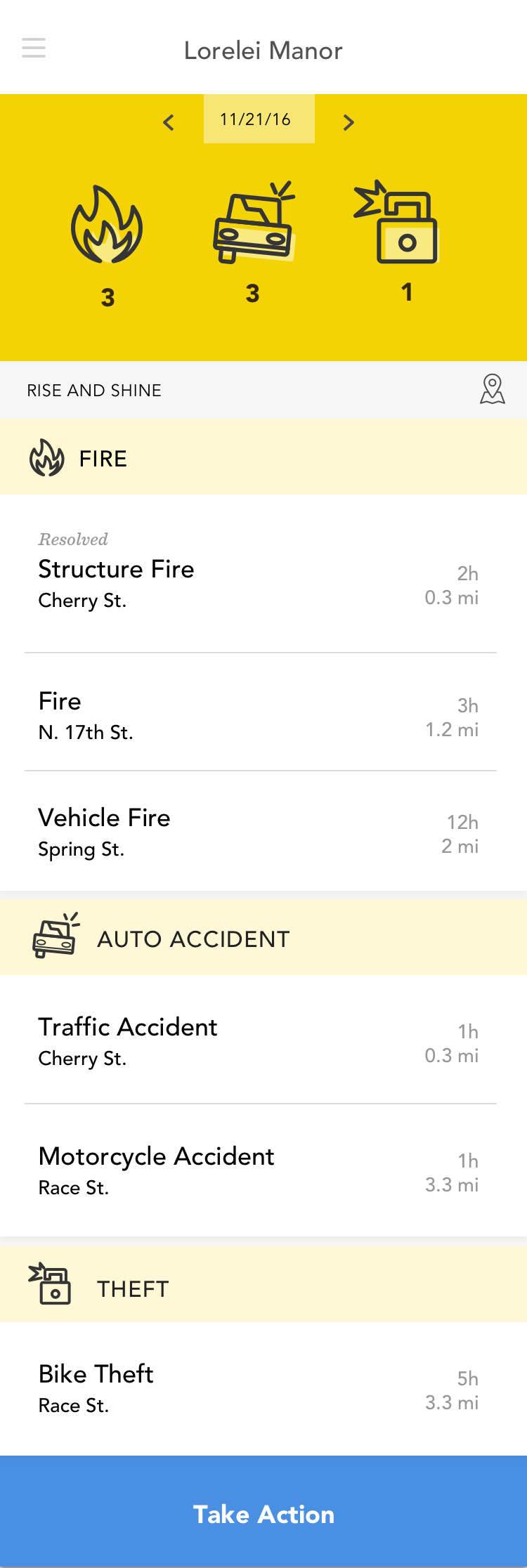This is a detailed and cleaned-up caption for the given screenshot:

---

The image is a portrait-oriented screenshot displaying various elements and information. In the top left corner, there are three light gray horizontal lines, typically indicative of a menu icon. Centralized at the top, in bold black text, it reads "Lorelei Manor."

Beneath this title, a yellow rectangle features two sections. The upper portion, in a slightly lighter yellow shade, contains black text that displays the date "11-21-16." Directly below this, there are three icons with associated numbers:

1. A flame icon with the number "3" beneath it.
2. A car icon with just one tire, appearing tilted, also with the number "3" beneath it.
3. A lock icon with a flame above its left side and the number "1" below it.

Continuing below these icons, in bold black text, it declares "Rise and Shine."

Further down, there are various yellow boxes containing detailed information about recent incidents:

1. **Yellow Box 1:**
   - **Icon:** Fire icon
   - **Text:** "Resolved, Structure Fire, Cherry Street, 2 hours, 0.3 miles"

2. **Incident Rows:**
   - **Fire:** North 17th Street, 3 hours, 1.2 miles
   - **Vehicle Fire:** Spring Street, 12 hours, 2 miles

3. **Light Yellow Rectangle:**
   - **Title:** "Auto Accident"
   - **Details:** Traffic Accident, Cherry Street, 1 hour, 0.3 miles
   - **Details:** Motorcycle Accident, Race Street, 1 hour, 3.3 miles

4. **Yellow Box 2:**
   - **Title:** "Theft"
   - **Details:** Bike Theft, Race Street, 5 hours, 3.3 miles

At the bottom of the screenshot, there is a blue band featuring white text that urges action, reading "Take Action."

---

This enhanced caption provides a clear, comprehensive description of all elements present in the screenshot, detailing their positions, colors, and associated information.